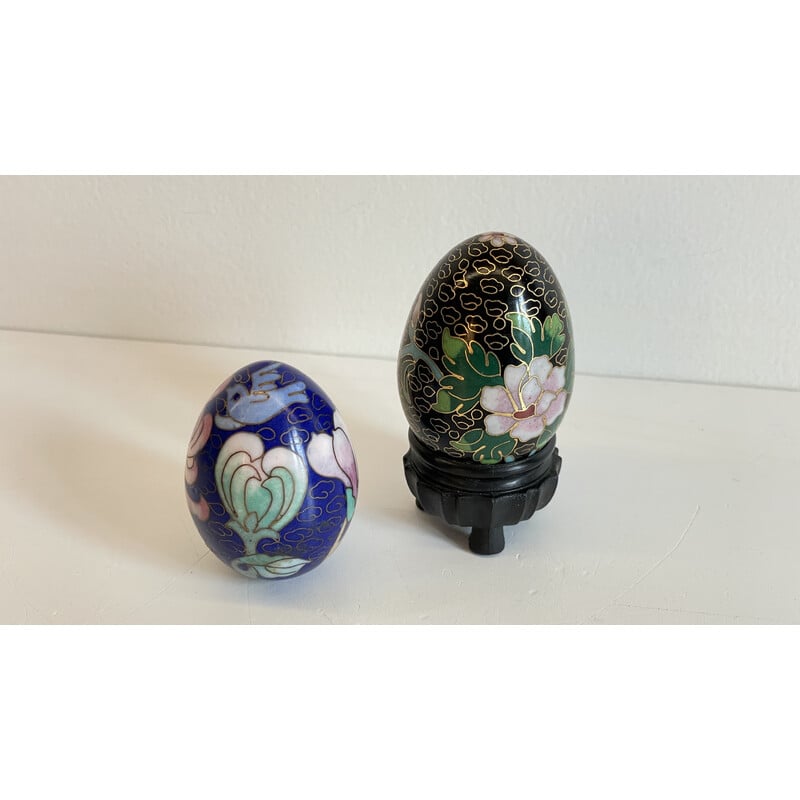This image is a detailed photograph of two intricately designed, decorative cloisonné eggs placed side by side on a beige table against a tan background. The egg on the left features a dark royal blue background adorned with gold lines forming abstract patterns, with delicate cloud-like shapes filled in gold. This egg also showcases a lighter shade of bluebird at the top, surrounded by pink, green, and white flowers. The egg on the right stands on a black base and is primarily black with similar gold abstract shapes. At its center is a prominent pink and white flower, with green leaves, all outlined in gold. Both eggs sit approximately an inch apart, diagonally positioned at the center of the table, displaying an exquisite blend of vibrant colors and fine art details.